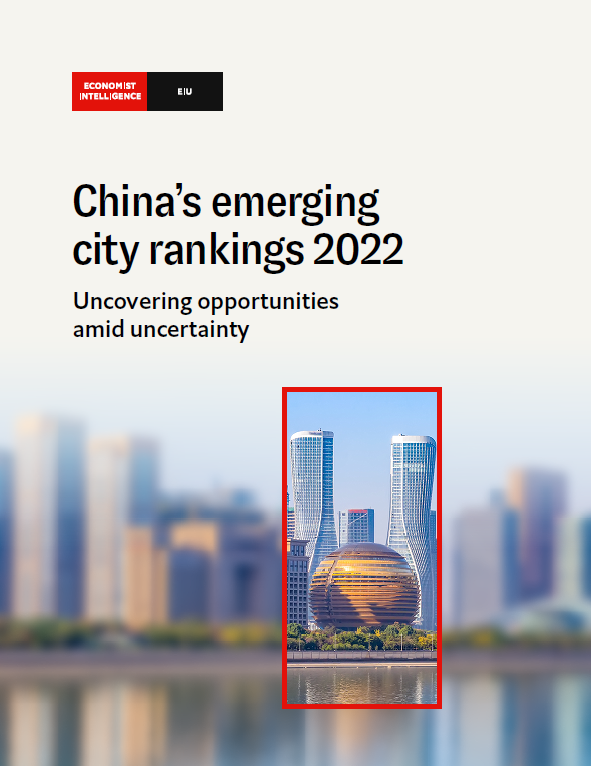The image appears to be the header for an article on a website. The background transitions from a grayish light blue color at the top to a more detailed urban scene at the bottom, showcasing a cityscape with tall skyscrapers. At the very bottom, there is a pond or river area flanked by trees, adding a natural element to the urban setting. 

Central to the image are two skyscrapers that have been highlighted within a red box. Inside this red box, there is a conspicuous gold and golden-brown orb-like building with a brown top. Flanking this structure are two tall skyscrapers, one on the left and one on the right. Nestled between these skyscrapers is a smaller, gray building, which features a red section on its roof.

The upper left corner of the image features a red and black half-and-half label reading "Economist Intelligence." To the right of this label is another text block that reads "EU." Below this, the title "China's Emerging City Rankings 2022: Uncovering Opportunities Amid Uncertainty" is written in black text.